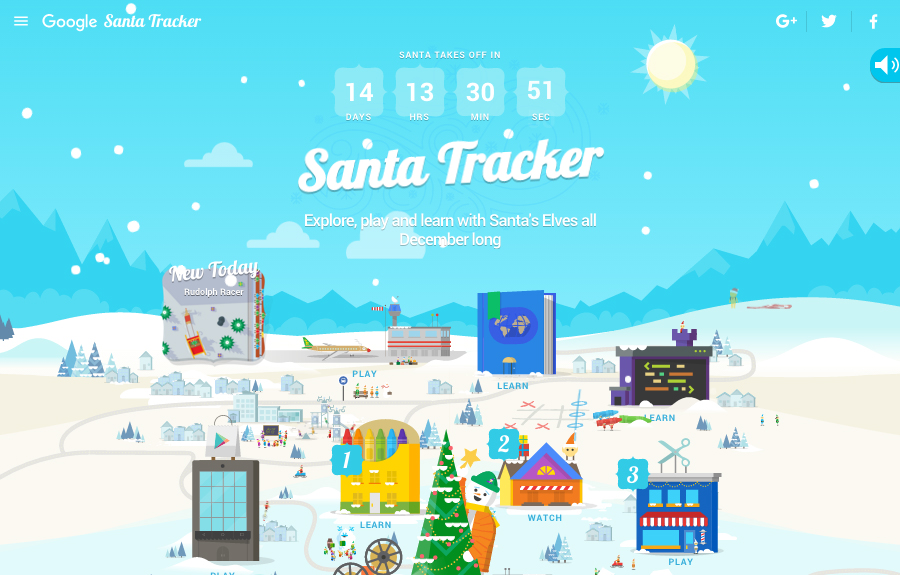This image depicts Google's Santa Tracker interface, a whimsical and festive countdown to Santa's departure. 

At the top left corner, three white lines form a drop-down menu icon. To the right, the word "Google" is presented in white, with "Santa Tracker" written next to it in a bold cursive font. Centrally located, the phrase "Santa Takes Off In" is rendered in small white capital letters. Below this, four distinct blocks resembling ice cubes display a countdown: "14" for days, "13" for hours (HRS), "30" for minutes (MIN), and "51" for seconds (SEC). These blocks feature a transparent blue background with white text.

To the right of the countdown is an illustrated sun. The lower left corner features clouds and snowflakes, while dark blue mountains span the middle of the page. Various clipart-style books, presents, and buildings are scattered across the scene, some labeled for emphasis. A yellow box of crayons, marked with a blue square and an italicized white character, stands out. Additionally, a building labeled with a "2" and another blue building labeled with a "3" are noticeable.

At the bottom of the countdown, a larger and slightly slanted "Santa Tracker" is written in a similar cursive font to the one near the logo, with an artistic tilt that has the "S" sloping down to the left and the "R" rising to the right. This charming and detailed visual encapsulates the festive spirit and playful nature of the Santa Tracker.